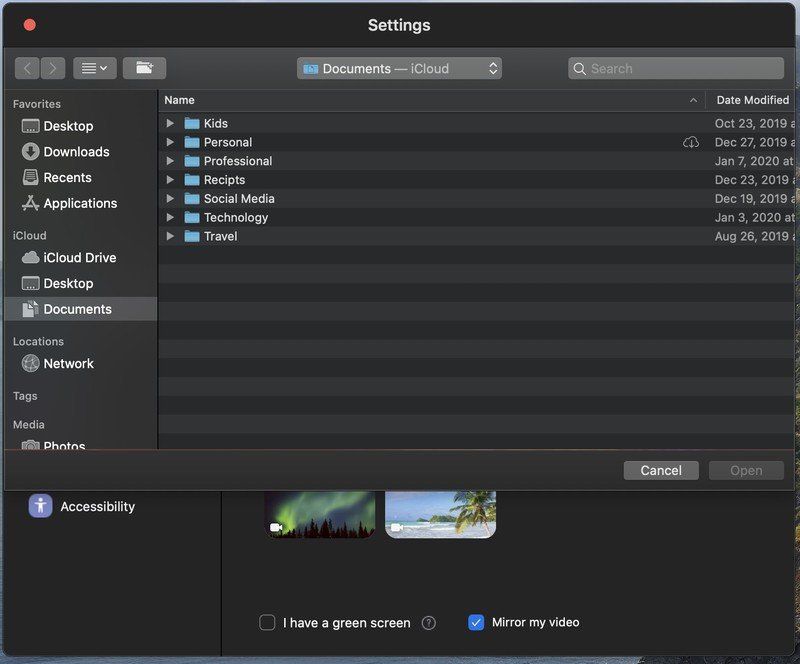The image displays a comprehensive view of a computer's file management system, featuring various directories and recent file modifications. Specifically, the left sidebar outlines several main folders and categories, including iTunes, Desktop, Downloads, Recents, and Applications. Within the iCloud section, subfolders such as iCloud Drive, Desktop, Documents, Network, Photos under Media, and Network are prominently listed. The iCloud folder further categorizes files into subfolders like Documents under iCloud, Kids, Professionals, Receipts, Social Media, Technology, and Travel. Each folder appears to have been modified on distinct dates - notably, 1st October 2019, 2nd December 2019, 3rd January 2020, 4th December 2019, 5th December 2019, 6th January 2020, and 7th August 2019.